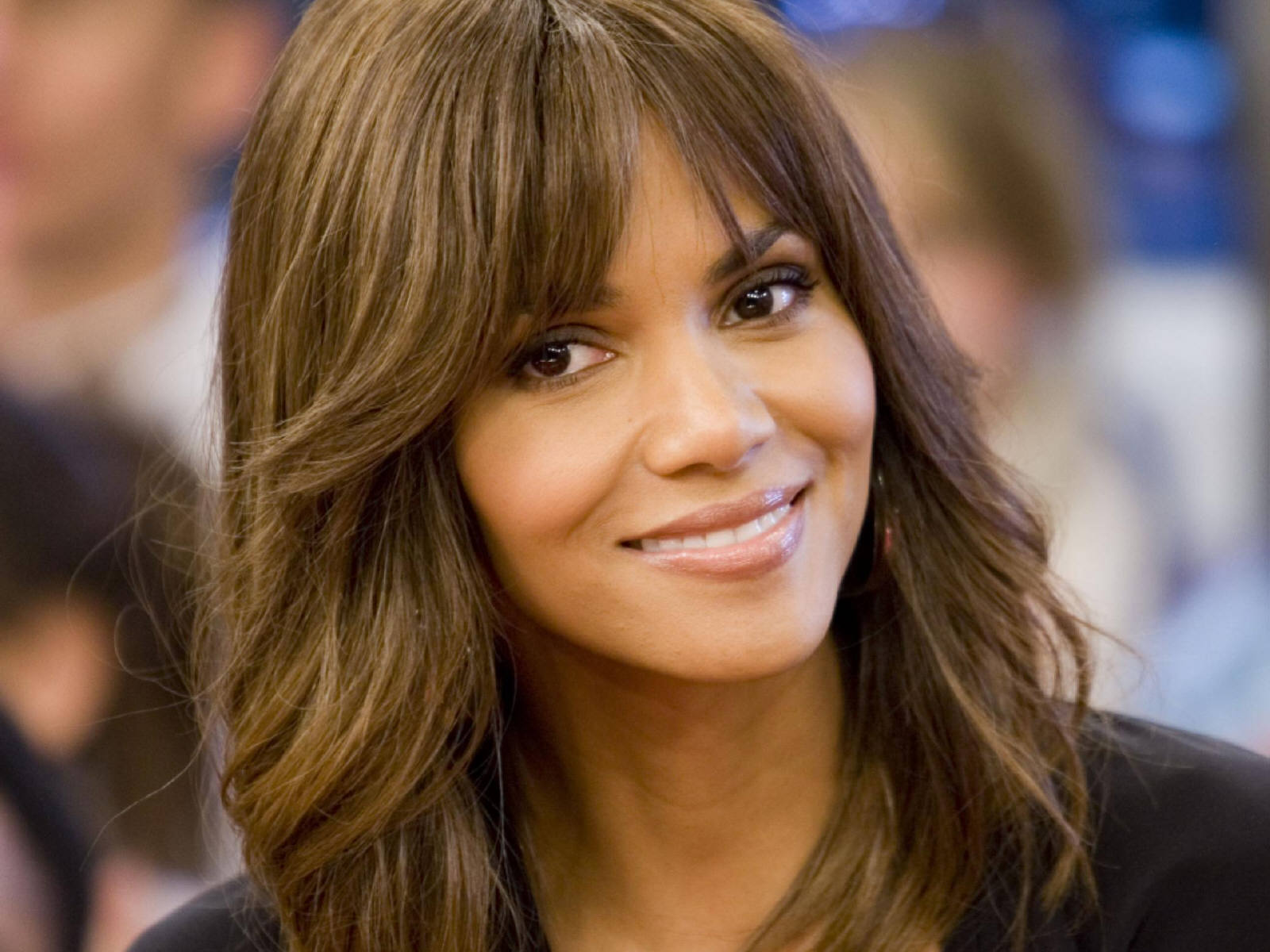This is a detailed close-up photo of Halle Berry, or someone who closely resembles her, likely taken at a public event given the presence of blurry figures and diverse background colors such as blue, white, black, and flesh tones. Halle Berry's hair, a rich chocolatey brown with lighter highlights, extends slightly past her shoulders and partially obscures her black jacket or knit shirt. Her head is slightly tilted to the left, which might be due to the angle of the photograph. Halle Berry's expressive face features dark brown eyes, shiny lip gloss, and slightly open lips revealing her bright white teeth beneath a soft smile. The overall composition and background elements suggest a lively yet intimate moment captured with emphasis on her radiant and polished appearance.